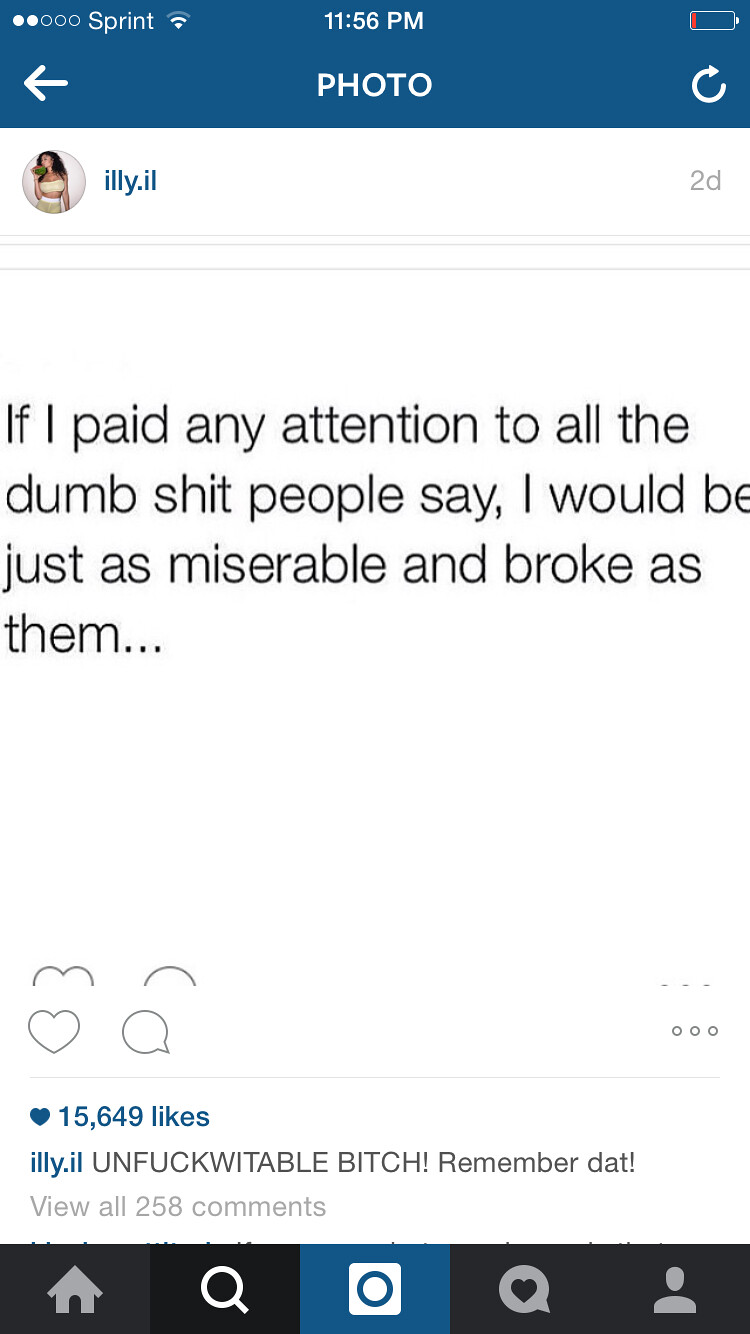This image appears to be a screenshot taken from a mobile phone, showcasing a social media post. The screenshot captures the phone's interface with blue across the top, featuring the time "11:56 p.m." and indicators for battery, Wi-Fi, and the network provider Sprint. Just below, the word "Photo" is displayed, suggesting that this is an image from the camera roll.

The main content features a profile photo of a woman, next to the username "ILLY.IL" on the upper left. To the right of the username, it states "2d," indicating that the post was made two days ago. The central part of the image displays a quote in bold black text on a white background that reads: "If I paid any attention to all the dumb shit people say, I would be just as miserable and broke as them."

Below the quote, a heart icon signifies that the post has received 15,649 likes. Additionally, there is a balloon icon suggesting the possibility to comment. The first comment appears below these icons, reading: "ILLY.IL unfuckwittable bitch remember dat!" followed by an invitation to "View all 258 comments." At the bottom of the screenshot, icons representing the homepage, search, likes, and profile hint that this is likely an Instagram post.